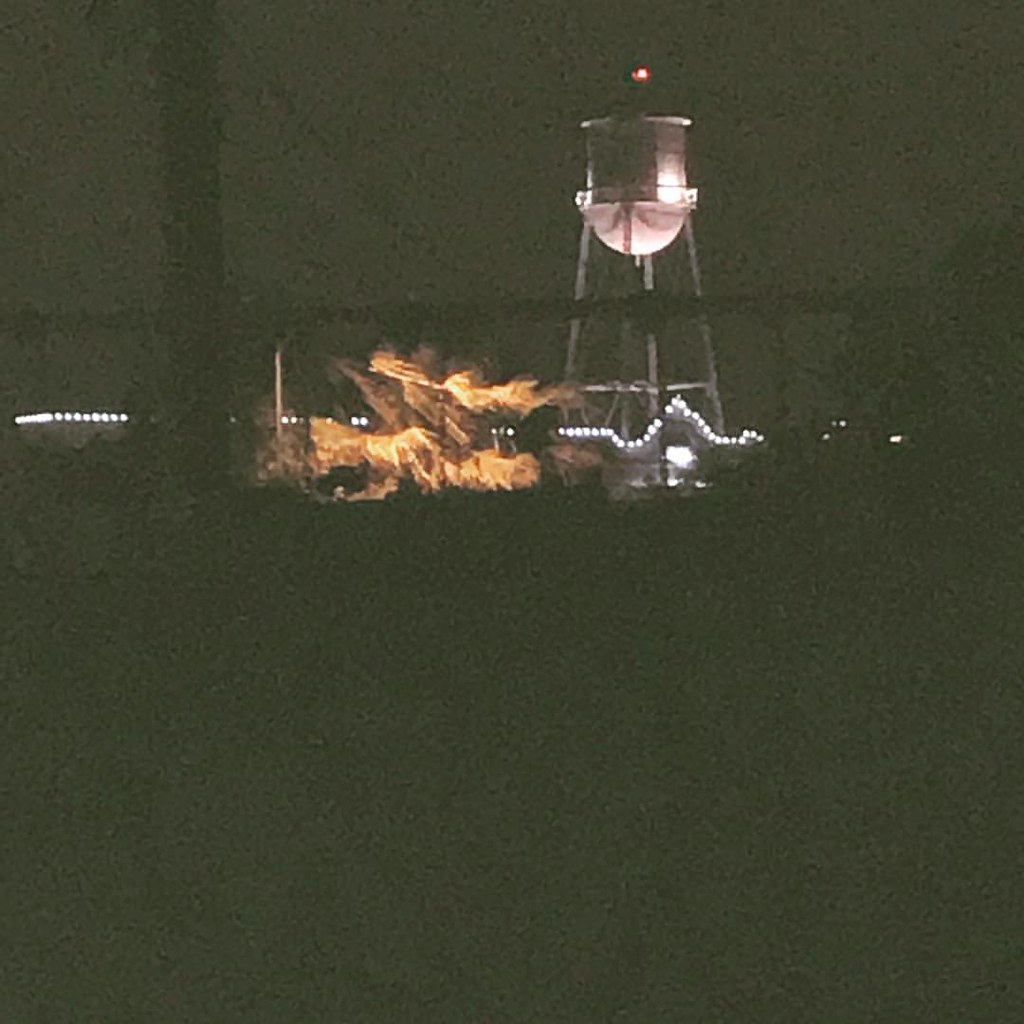In this nighttime, desaturated photograph, a prominently illuminated water tower stands as the central feature. The water tower, supported by four legs forming a sturdy base, has a round-bottom tank with a black top crowned by an orange-red light. Rows of white lights run vertically and horizontally across the structure. The background features interspersed lights that might belong to a building or a long pier, suggesting human activity beneath the tower. Black lines run both vertically and horizontally alongside the tower, adding structural depth to the image. Notably, two flame-like patches of orange and black appear between the water tower and these black supports, enhancing the scene's enigmatic atmosphere. The entire bottom half of the picture is shrouded in darkness, bringing a stark contrast to the illuminated elements and making the tower's lit details stand out even more strikingly.